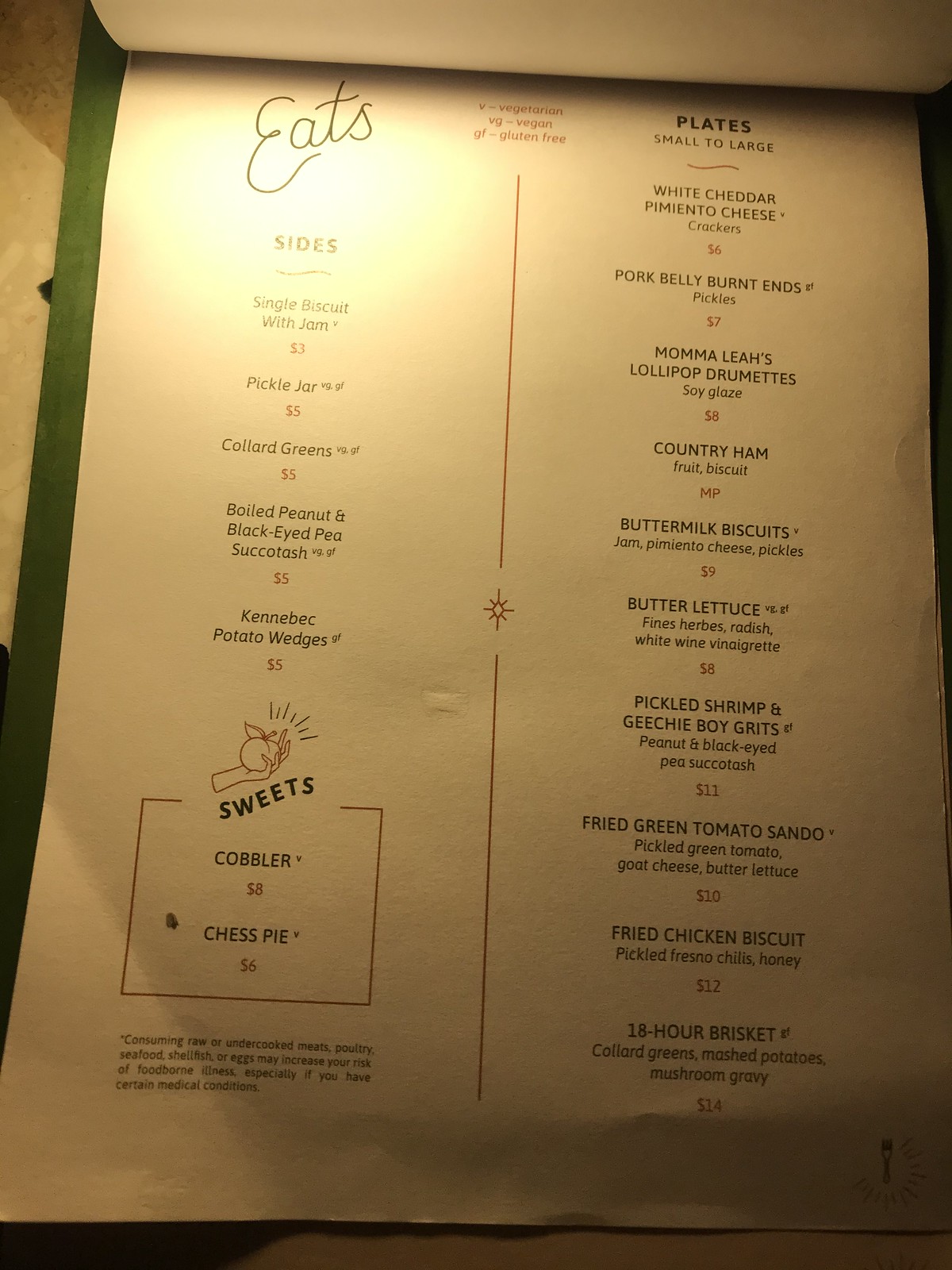The image showcases a vintage piece of paper with a tan background, mounted on a green diagonal strip visible on the left side. The paper has aged to a faded yellow hue, and features a slender red line running vertically down its center, creating two columns. The left column, labeled "Eats," lists about five items that are too small to read clearly, written in dark text. Near the bottom of this column, there is a sketch of a red hand holding a piece of fruit. Below this illustration, the word "Sweets" appears in bold black lettering, followed by legible menu items: "Cobbler" and "Chess Pie."

The right column begins with the heading "Plates" in black text. The menu items listed here, though partially readable, include: "White Cheddar," "Pork Belly," "Mama Lia's Lollipop Drumettes," "Country Ham," "Buttermilk Biscuits," "Butter Lettuce," "Pickled Shrimp," "Geechee Boy Grits," "Fried Green Tomatoes," "Fried Chicken Biscuit," and "18-Hour Brisket." The timeless design and hand-drawn elements give the menu a rustic and nostalgic charm.